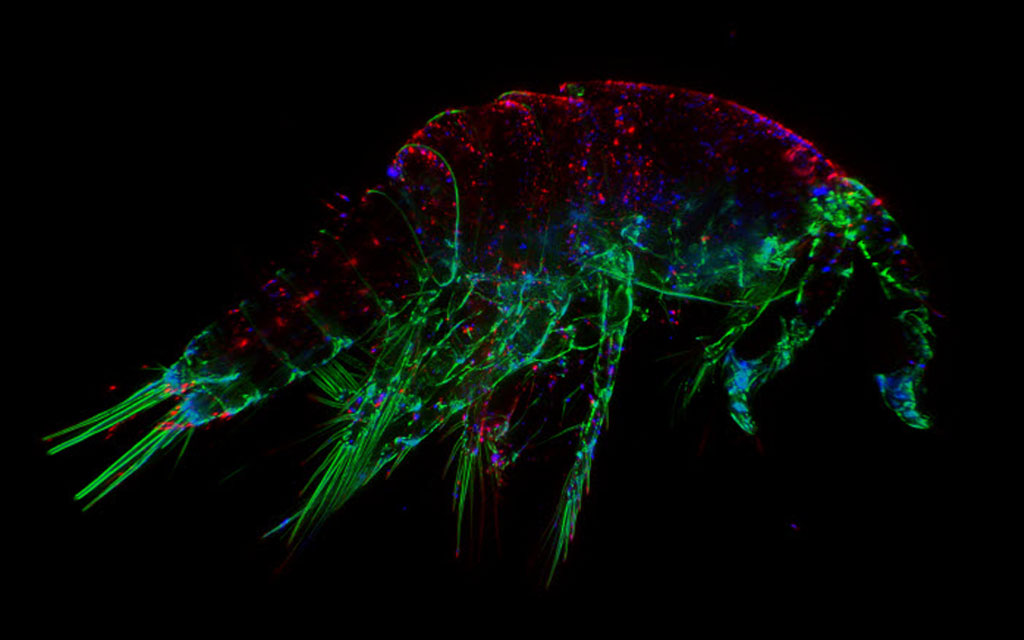The image shows a detailed X-ray of an aquatic creature, facing the left side, with a dark, black background. The upper part of the creature is illuminated with neon red, blue, and black lights, radiating from its rounded, shrimp-like body. This intriguing creature features two distinct sets of long, green-lit antennae sprouting from its head-like structure on the left. Along the entire length of its elongated body, there are a total of 92 long, vividly red legs, which are clearly visible beneath the brighter neon lights. The lower portion of the creature glows in vibrant green, highlighting the segmented appendages and spike-like parts that give it an otherworldly appearance. This captivating image distinctly features neon outlines and coloration, creating a surreal and detailed portrayal of the creature in its dark, aquatic environment.